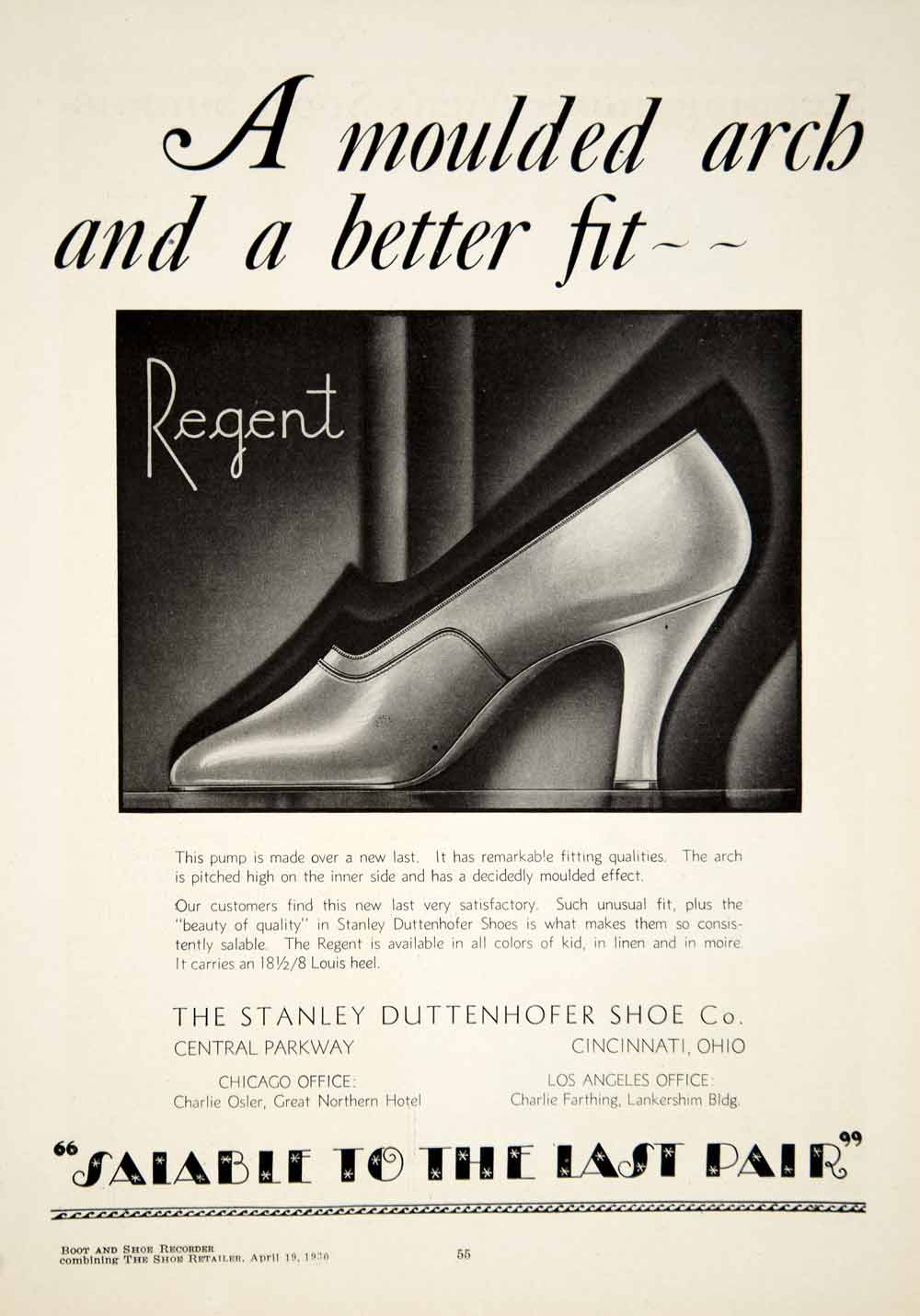This vintage advertisement from the Stanley Deutenhofer Shoe Company of Cincinnati, Ohio features a polished, silver-colored high-heeled pump shoe set against an Art Deco-themed background. At the top of the ad in bold black lettering, it proclaims "A Molded Arch and a Better Fit." The shoe is labeled "Regent" and is described in detail with text about its superior fit, attributed to its new last design. Below the image, the ad emphasizes that the shoes are "salable to the last pair." The background appears neutral, possibly white, aligning with the monochromatic color scheme typical of old magazine ads. Additional text reveals that the company has offices in Cincinnati and Chicago, indicating a broader market reach. The shoe itself stands out as an artistic focal point, appealing to shoe stores with its sleek design and comfortable fit.